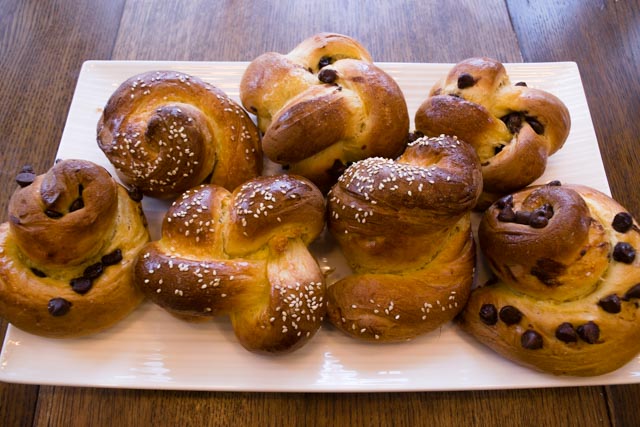The image captures a beautifully arranged offering of baked goods set on a wooden table during an office meeting. The wooden table is designed with three panels, and the dish is resting on the removable middle leaf that helps extend the table. The offering is presented on an elegant white rectangular plate with upturned edges. The plate features an assortment of delectable treats: on the far edges, there are four large, fluffy croissant rolls studded with chocolate chips, while the center showcases three impressive pretzels generously topped with sesame seeds. In total, there are seven mouth-watering baked goods, all of which look incredibly delicious.